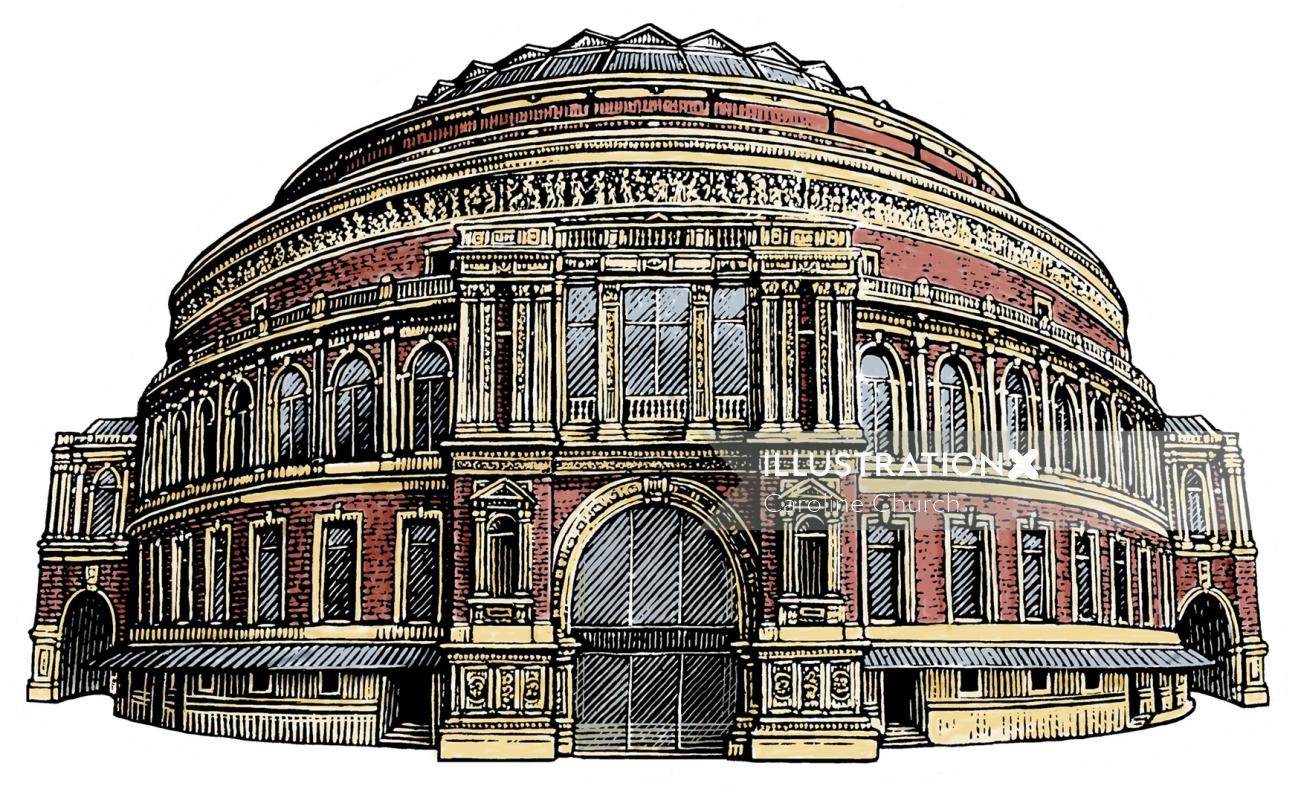This detailed illustration depicts a grand, round building with a domed roof, exuding a hand-drawn, almost cartoon-like artistry. The structure, colored predominantly in red brick with subtle gold hues, showcases intricate architectural details. The façade features a semi-circular, protruding front section flanked by two side buildings, each with archway walkways allowing entrance. The front of the building is ornamented with decorative brickwork forming half-rings and includes a prominent large archway window that spans the first and second floors at the center. Additionally, the building, standing between two and four stories high, has an assortment of windows; some on the ground floor are square-topped, while others are elegantly arched. The windows and doors display distinctive diagonal black and white lines. Statuettes embellish the top rim of the dome, adding to its classic charm. Overlaying the building, a watermark reads “ILLUSTRATION X CAROLINE CHURCH,” with "ILLUSTRATION X" bolded in white, located off-center to the right. The backdrop of this striking image is a pure white color, further emphasizing the building's detailed design elements.